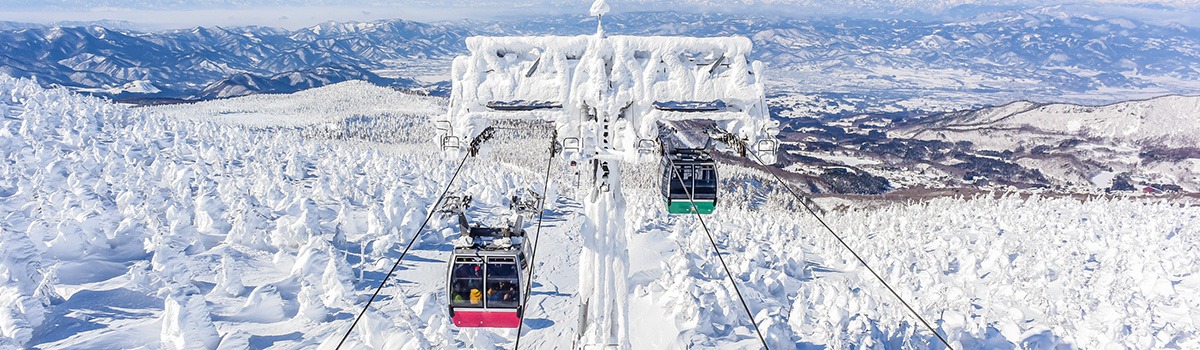A breathtaking photograph showcases a winter wonderland with two gondolas traversing a snowy landscape. The gondola on the left, adorned with a red bar across its white cabin, is approaching the camera, while the one on the right, featuring a green bar, recedes into the distance. They glide above a dense blanket of snow-covered trees, their shapes almost indistinguishable beneath the heavy snow accumulation. The ground below is similarly covered, with shadows cast by the trees indicating it's a sunny day. In the background, a series of steep mountain ranges transitions from dark gray to light gray and white, creating a dramatic contrast against the slim sliver of sky at the top of the image. The entire scene exudes the tranquility of a freshly snowed-in landscape, with subtle hints of black earth peeking through a lower valley, adding depth to this serene winter tableau.